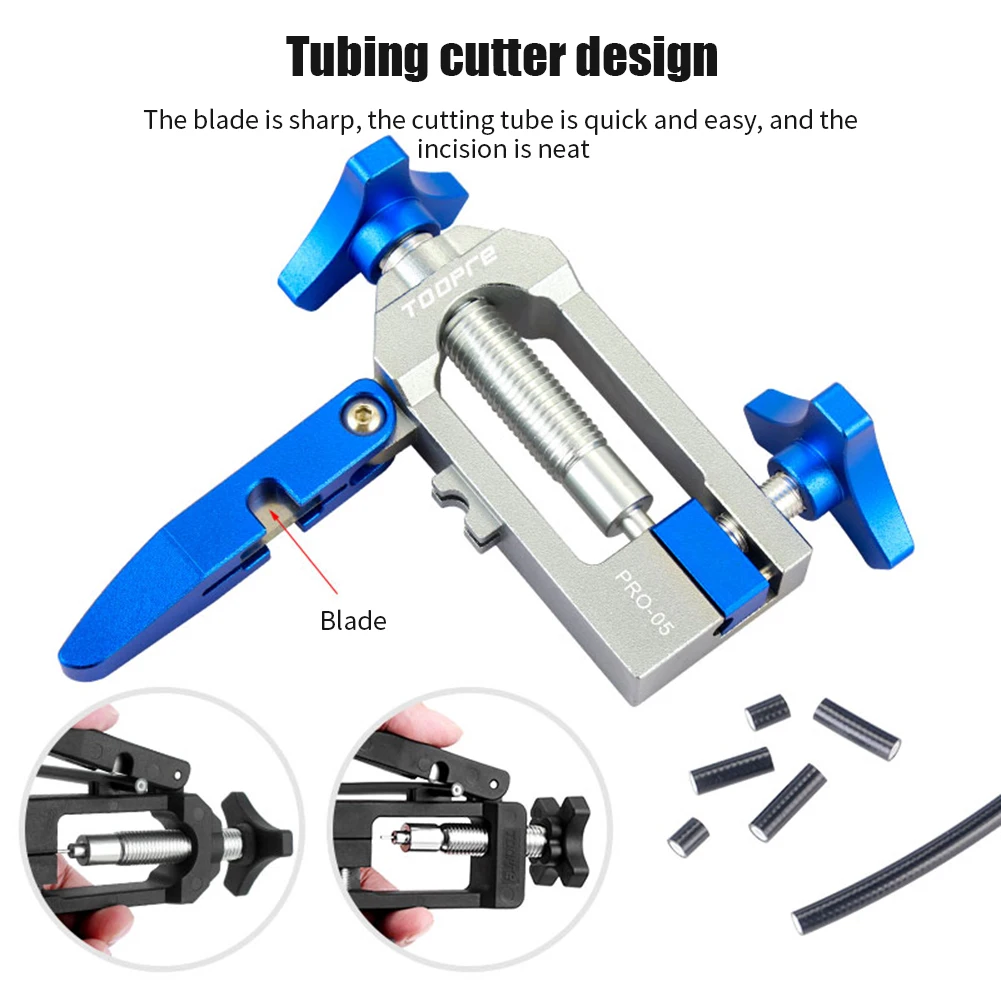The image depicts a detailed advertisement for a tubing cutter design tool. At the top, bold blocky text reads "Tubing Cutter Design," followed by the description: “the blade is sharp, the cutting tube is quick and easy, and the incision is neat.” The showcased tool features real photos, not illustrations, emphasizing its practical use. The cutter itself is primarily silver with blue handles and fixtures. It includes a blade extending at a 45-degree angle and is equipped with two blue, rotatable points for adjustments. One blue handle is on the top right of the silver case, which includes a central screw, while another blue area for adjustments is above the blade on the top left. At the bottom left of the advertisement, there are two inset circles displaying interchangeable attachments for the tool, indicating its versatility. The bottom right corner shows small, scattered tubing pieces of various sizes that the cutter cleanly severed, demonstrating the device's ability to handle different diameters. Additionally, there is a label identifying the brand as "Tupre Pro-05" with a red arrow pointing to the blade, and an image of a person using the cutter. The entire setup is designed to highlight both the functionality and efficiency of the tubing cutter.